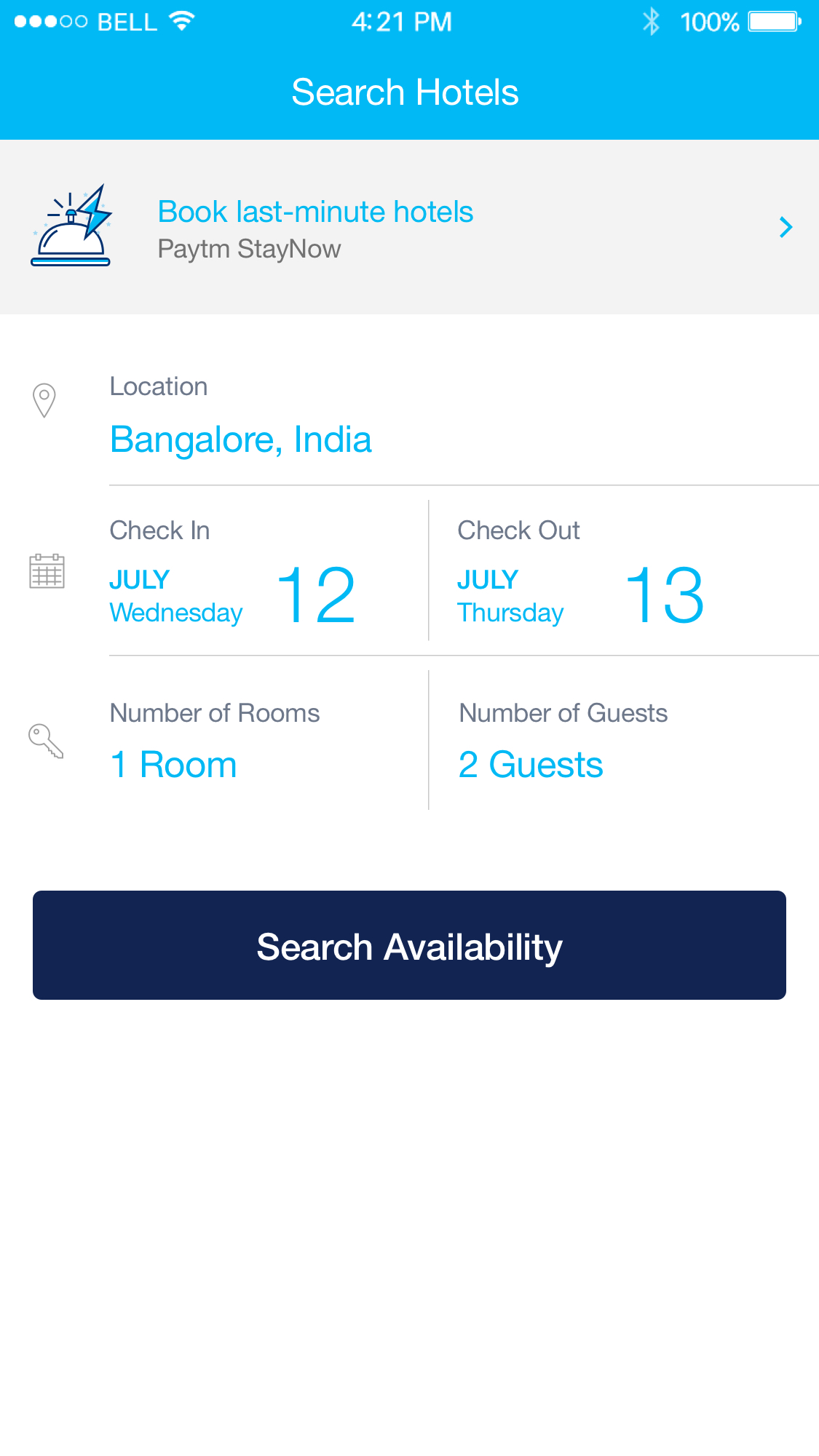This image is a screenshot of a hotel booking application's interface. At the top of the screen, enclosed in a light blue rectangular bar, various status icons are displayed, including a bell indicating three out of five bars of reception, a Wi-Fi icon showing the connection status, the current time which reads 4:21 p.m., and a battery icon at 100% charge. The text "Search Hotels" is prominently displayed.

Below this, on a white background, bold blue and black text reads "Book Last-Minute Hotels" and "PayTM, Stay Now." Adjacent to this text, on the left side, is an illustration of an old-fashioned desk bell.

Further down, the location is specified as Bangalore, India, with check-in and check-out dates listed as Wednesday, July 12th, and Thursday, July 13th, respectively. These dates are accompanied by an illustrated calendar icon positioned to their left.

Below this section, an illustration of a key denotes the booking details: "Number of rooms: One room" and "Number of guests: Two guests." Finally, at the bottom, there's a button labeled "Search Availability," inviting the user to proceed with finding available rooms.